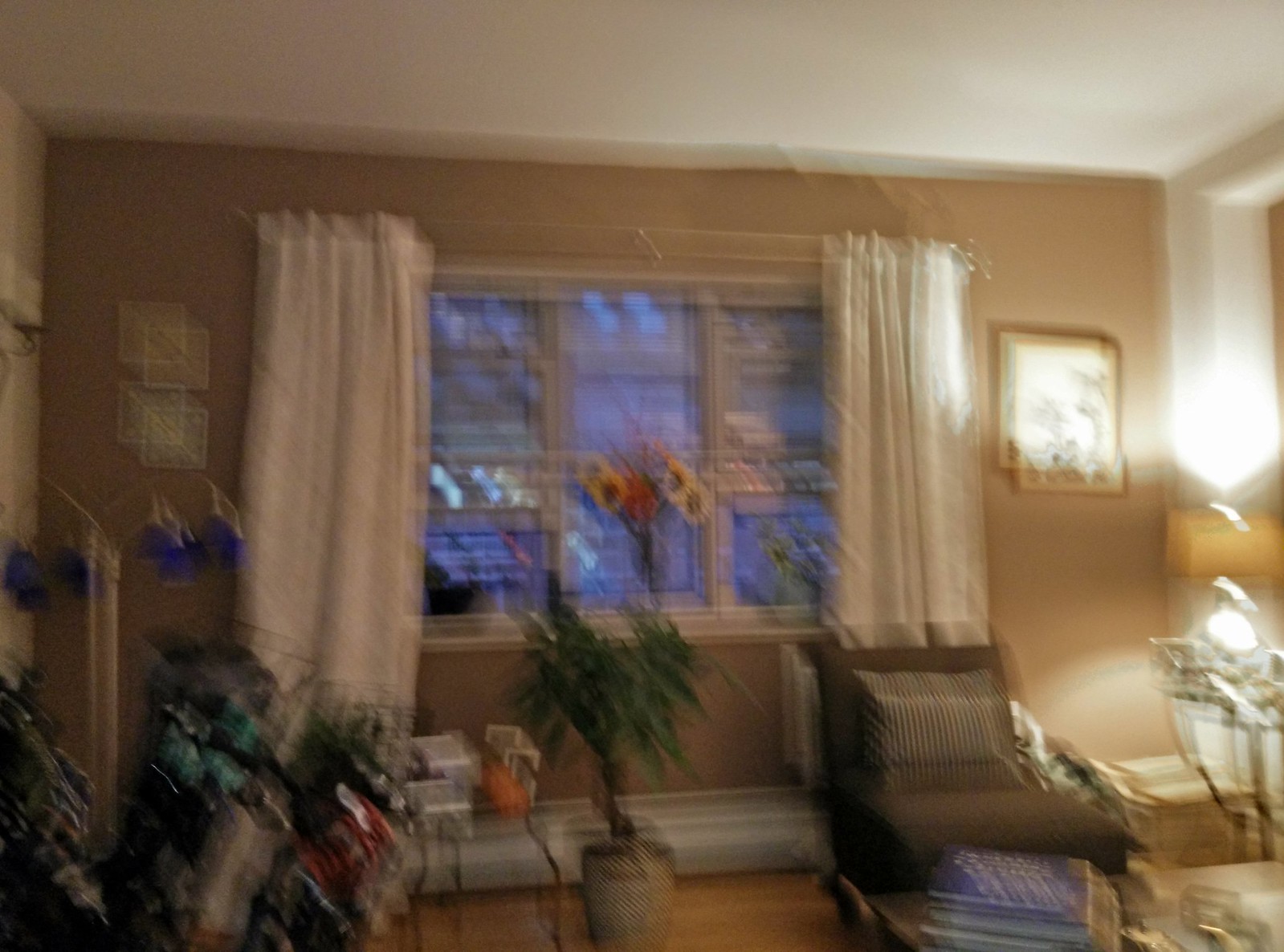This is a very blurry, rectangular landscape image of a living room. The back wall, a light brown or coffee color, features a very large landscape window with off-white curtains partially pulled back, revealing multiple individual window panes. The scene outside appears blue but is indistinct due to the blurriness. A transparent vase with sunflowers and a few other flowers sits on the lower windowsill. On the right side of the window hangs a picture, while two smaller pictures adorn the left. 

In front of the window, there's a potted plant with green leaves in a large, grayish pot, standing about four feet tall, its wooden stem thick and strong. To the right of this plant is a single brown-cushioned chair facing the viewer, with what appears to be a Lazy Boy chair adjacent to it. A glass-topped table sits near the chair with a lamp on it. The lamp, possibly lacking a shade, shines brightly and illuminates much of the room, contributing to the overall light. The lower left corner is darker and messier, its details obscured by the blurriness of the image.

The ceiling is partially visible and white, while the floor appears to be medium wood-colored paneling or tiled.